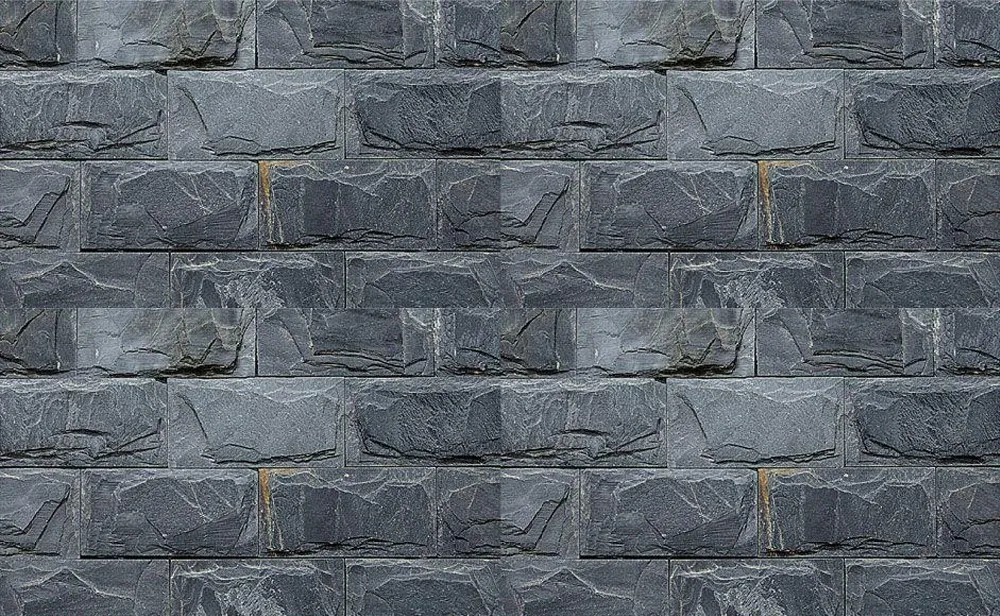This is a detailed photograph of a stone wall constructed from gray concrete bricks, arranged in a typical masonry pattern. Each brick is a horizontal rectangle, and the bricks are stacked in an alternating pattern where the middle of one brick aligns with the ends of the bricks above and below it. The bricks vary in color, displaying a range of gray tones from light to dark, with occasional pops of white and a notable copper-colored staining on one of the lower bricks. The surface of the bricks is rough and textured, featuring lines and wrinkles that give them a distinct, non-uniform appearance. The wall appears to be composed of many individual bricks—around 30 or 40—each contributing to the alternating pattern. The image itself may be duplicated to form a larger single picture, as suggested by the recurring patterns and a central point where bricks seem almost mirrored. This structured repetition and the intricate detailing on the bricks lend the wall a unique, almost marble-like aesthetic.